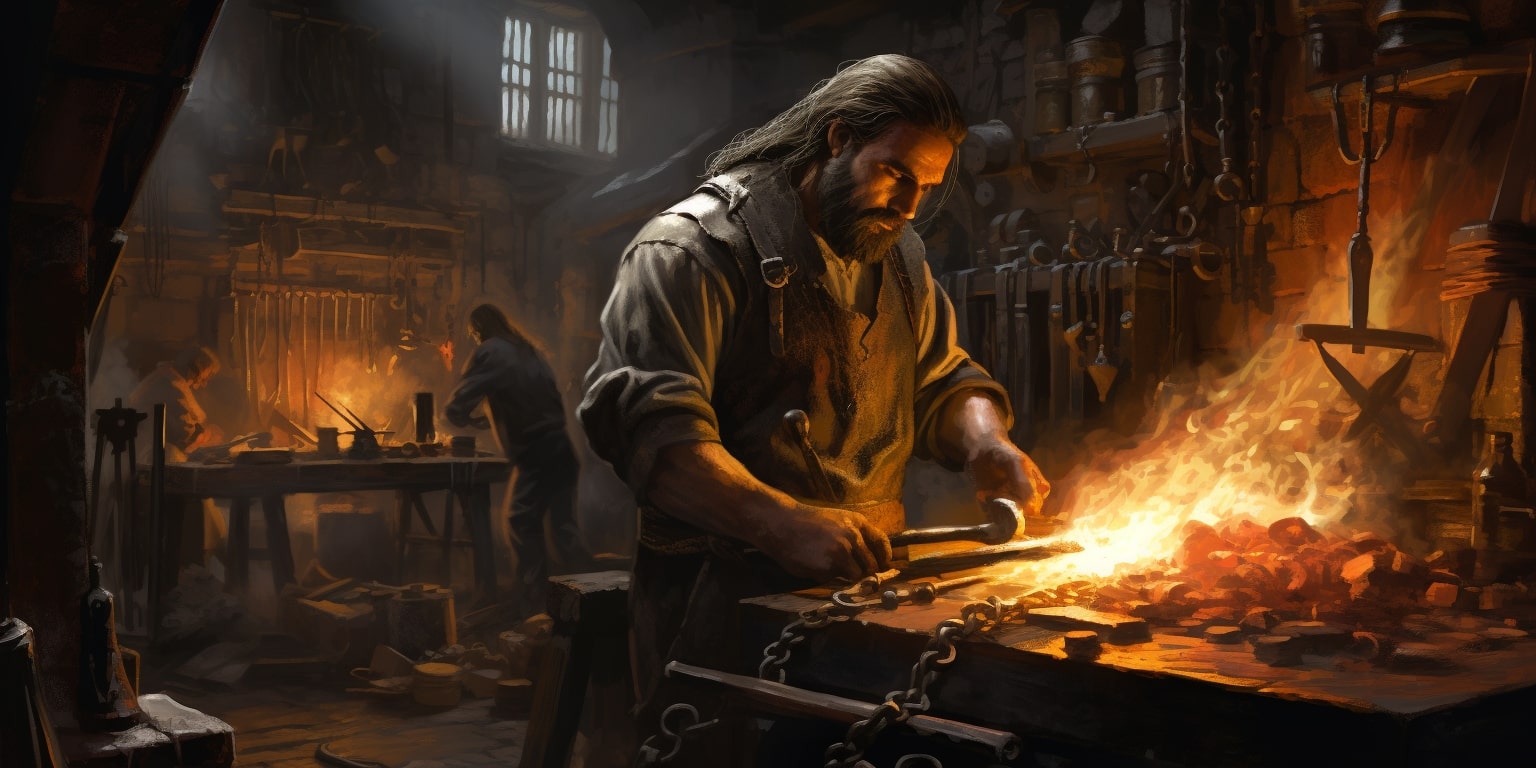The 3D color illustration, possibly an AI rendering, depicts a medieval blacksmith's workshop in landscape orientation. The central figure is a white man with long brown hair and a beard, wearing a dark brown leather apron with buckles and rolled-up sleeves. He is intensely focused on his work at a dark wood table angled to the bottom right, where he is possibly grinding a metal weapon on a stone, sending yellow sparks and flames to the right side. In the dimly lit workshop, characterized by its brick walls adorned with various metal tools, there are additional figures visible in the background, similarly engaged at tables with flames, contributing to the fiery ambiance. A barred window at the top left filters in a small amount of light, adding to the room's dark interior, enhancing the old-school fantasy setting of the entire scene.